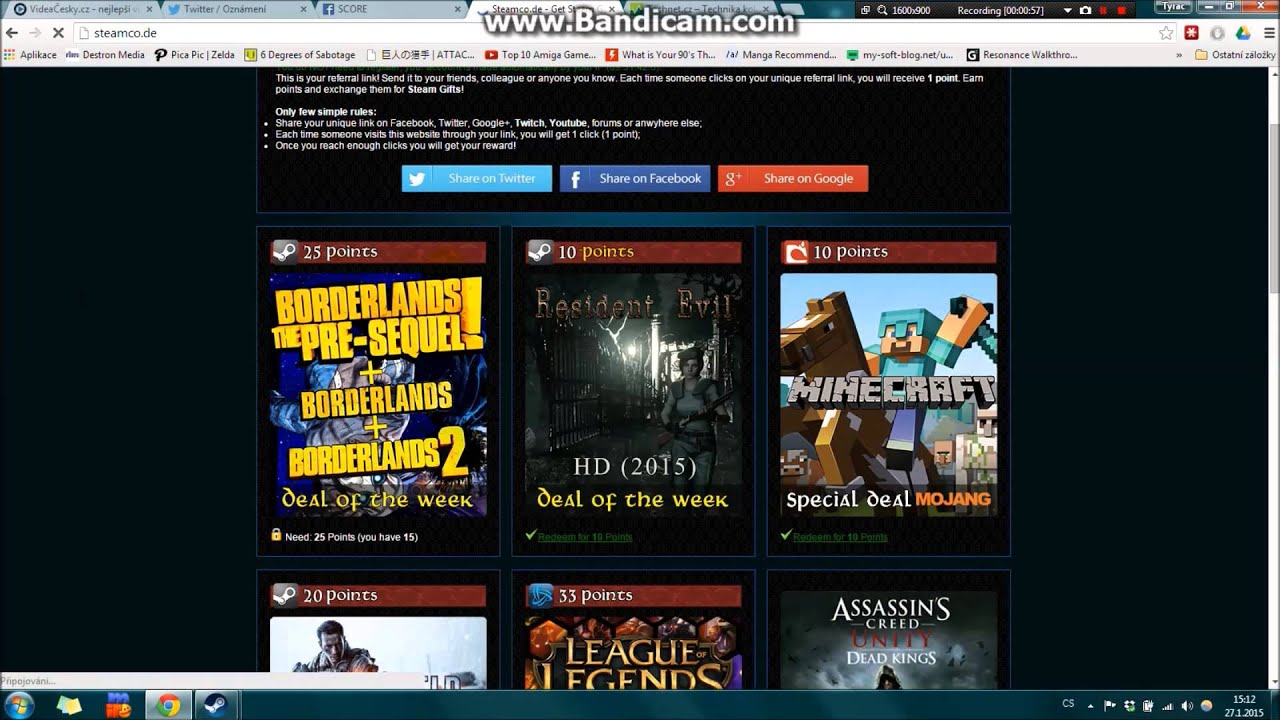The screenshot captures a Windows desktop with an open browser displaying the Steamcode.de website. Along the top of the browser window, there are inactive tabs for Twitter and Facebook. The user is recording their screen, as indicated by a recording bar showing options to record, stop, and take a screenshot, prominently visible. A watermark from Bandicam, located at the top center, reads "www.bandicam.com."

The website features a dark blue background with darker blue and black boxes outlined in a slightly lighter blue, making them stand out. The text is in white, and there are buttons for sharing content on Twitter, Facebook, and Google. The visible portion of the webpage displays several game posters with corresponding points. Notably, the top row showcases "Borderlands: The Pre-Sequel," "Borderlands," and "Borderlands 2," worth 25 points in total. There are six game posters in total, though the bottom row is partially obscured and not fully visible.